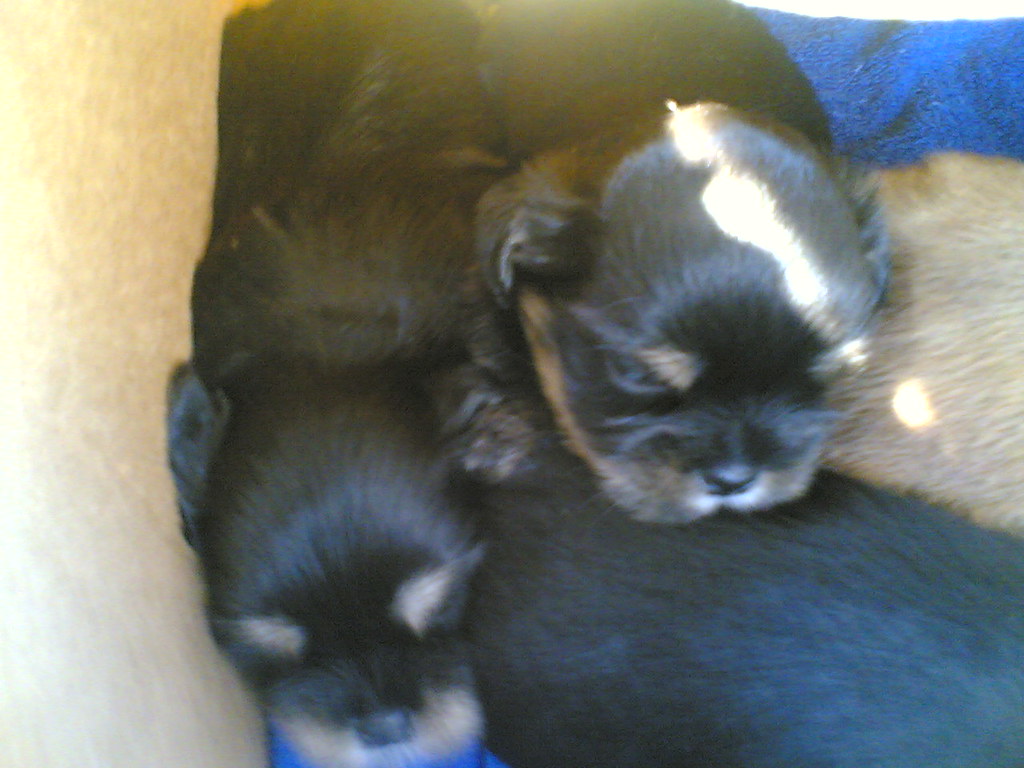The image is a close-up photograph capturing an endearing scene of at least three black-furred puppies, possibly resting in a box. The photograph is about 30% wider than it is tall, and it showcases the puppies nestled together, suggesting intimate proximity. Two of the puppies are distinctly visible, facing a position akin to six o'clock, while a third puppy's body is discernible, oriented roughly towards the upper left-hand corner or 10:30 position. These little ones have dark coats with distinctive light brown markings around their noses and above their eyes, with the rightmost puppy's head highlighted by a sunbeam.

The setting includes a mix of textures and items, indicating a cozy, makeshift bedding area. The left side features what appears to be a brown piece of cardboard, and the upper right side is occupied by what seems to be a blue towel or blanket. The bottom of the image shows some off-white fur, likely from their mother, lending to the snug atmosphere. The central part of the photograph is densely packed with dark fur, potentially suggesting the presence of another puppy or simply the puppies’ fur intertwined. Despite the slight blurriness and close-up nature of the photo, the puppies' cuteness and the intimate feel of their resting spot are clearly conveyed.